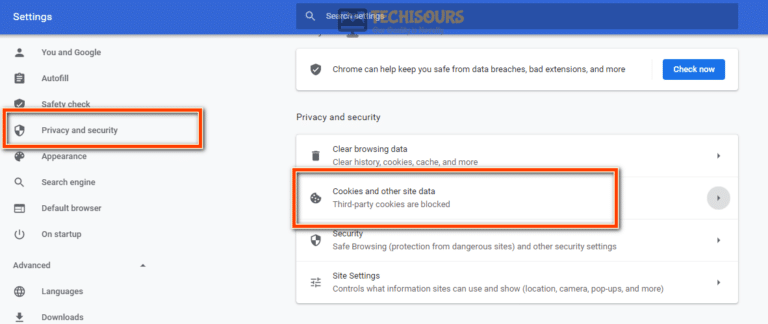This is a landscape-oriented partial screenshot of a website's settings page. The image is slightly low in resolution but remains perfectly visible. The top of the page features a blue border with the word "Settings" in white text on the left. In the middle of this border is a darker blue box that serves as a search bar, containing the phrase "Search settings" in white text and a search icon to its left. Superimposed in an opaque orange color over this search bar is the phrase "tech is sours."

The rest of the page has an off-white background. On the left is a vertical menu list featuring several sections, each with an appropriate icon and grey text. The sections from top to bottom are: "You and Google," "Autofill," "Safety check," and "Privacy and security," which is distinguished by an orange border box. Following these are "Appearance," "Search engine," "Default browser," and "On startup." Below these is a new section titled "Advanced," containing "Languages" and "Downloads," at which point the screenshot cuts off.

To the right of this menu, occupying two-thirds of the webpage, is the "Privacy and security" settings page. This section features a white box listing several options under the title "Privacy and security." The first option is "Clear browsing data," with a description underneath that reads, "Clear history, cookies, cache, and more," in grey text. The second option is "Cookies and other site data," which is accompanied by, "Third-party cookies are blocked," also in grey text and highlighted with a bright orange border box. 

Following this is the "Security" section, stating, "Safe browsing," with a description in brackets: "Protection from dangerous sites," followed by "and other security settings." The final option listed is "Site settings," which offers "controls of what information sites can use and show," including information like "location, camera, popups, and more," also enclosed in brackets.

At the top of this page is a small white box containing a message: "Chrome can help you keep safe from data breaches, bad extensions, and more." To the right of this message is a blue "Check now" button with white text.